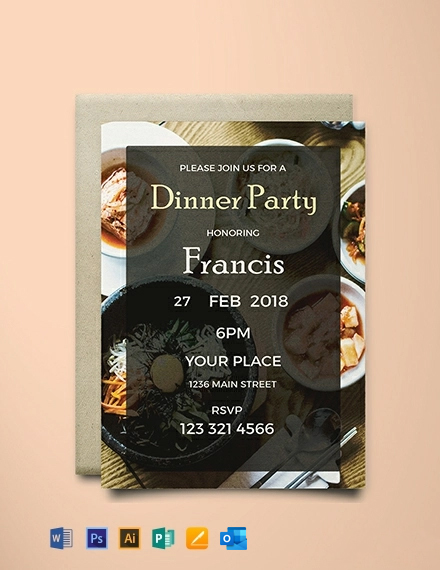In the image, there is a dinner party invitation prominently centered against a peach-pinkish beige background. The black invitation, which has a transparent quality, allows the underlying image of a table laden with various food items to peek through. It is slightly overlapping a tan envelope. The invitation is bordered with a design mimicking a food setting arranged around the table. The text on the invitation reads, "Please join us for a dinner party honoring Francis. 27th, FEB, 2018, 6 PM, Your Place, 1236 Main Street. RSVP 123-321-4566." The background of the image includes several computer window icons, such as those for Microsoft Word, Adobe Photoshop, Adobe Illustrator, Apple Pages, Microsoft PowerPoint, and Microsoft Outlook, suggesting that the invitation is a digital template still being edited. The color palette in the image features shades of beige, white, orange, red, and tan, contributing to a warm and festive atmosphere.